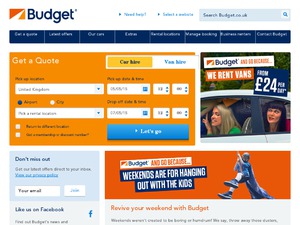A screenshot of a budget management screen featuring various UI elements:

- The top-left corner prominently displays the company's logo.
- To the right of the logo, in large blue letters, is the title "Budget."
- On the right side, there are two small, somewhat blurry blue buttons with unclear text, followed by a blue search bar equipped with a magnifying glass icon on the right.
- Below this, a dark blue horizontal rectangle runs across the screen, containing white menu items separated by vertical light white lines, although their text is illegible.
- To the left beneath this, there's some white space leading to an orange rectangle. Within this orange rectangle, "Get a Quote" is written in orange in the top-left corner.
- Adjacent to this, two buttons are placed: a yellow button on the left reading "Car" (with an unreadable second word) and a white button on the right with "View Here" written in blue.
- Below these buttons are two horizontal lines, each containing four drop-down boxes, intended for making car reservations. 
- At the bottom-right corner within this section is a blue "Let's Go" button.
- To the right of the orange rectangle, there is a square photo with the text "Budget. We rent vans," depicting women inside a car.
- In the bottom-left corner of the image, there is a blue box containing the text "Don't Miss Out," followed by two lines of smaller text, a white rectangular box labeled "Your Email," and a button to the right of it.
- Further to the right is another orange rectangle featuring an image on the right side, and on the left, it reads "Weekends are for hanging out with the kids."